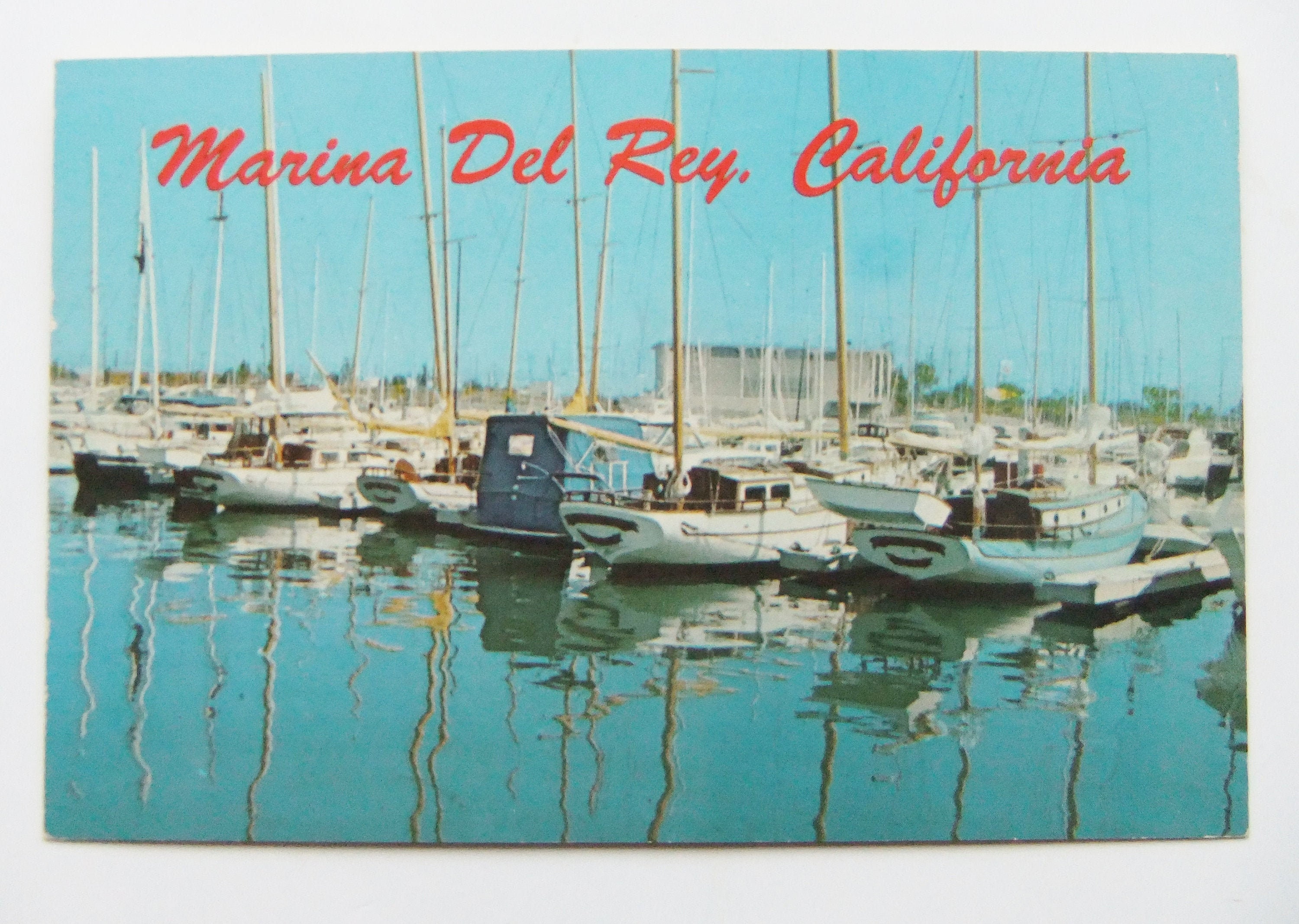This detailed image is a vintage postcard showcasing Marina del Rey, California, as indicated by the cursive red text at the top. The scene features a large dock populated with boats, primarily white, with a notable light blue and dark blue boat prominently positioned in the center. The boats, equipped with tall poles for sails, are neatly docked in their parking spots. The clear blue water creates a striking mirrored reflection of the boats, enhancing the picturesque quality of the scene. The sky is a vibrant blue, devoid of clouds, contributing to the serene and timeless feel of the image. In the distant background, a light brown rectangular building, possibly a hotel, and green trees frame the harbor, emphasizing the vintage aesthetic likely from the 1960s or 1970s. The overall style, colors, and composition evoke a sense of nostalgia, characteristic of postcards from that era.